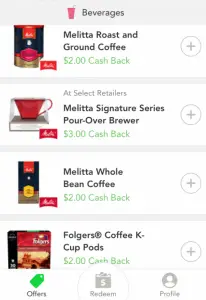### Caption:
Screenshot of an e-commerce app screen showcasing deals on beverages. The interface follows a minimalist design with alternating shades of gray rows highlighting each product. At the top, the title "Beverages" is prominently displayed, accompanied by a cute red icon of a drink with a straw on the left. Below the title, various coffee products are listed along with cashback offers. The products include:
- Melitta Roast and Ground Coffee with a $2 cashback offer available at select retailers.
- Melitta Signature Series Pour-Over Brewer offering a $3 cashback deal.
- Melitta Whole Bean Coffee eligible for a $2 cashback.
- Folgers Coffee K-Cup Pods with a $2 cashback incentive.

Each product entry features a small, circular button with a gray outline and a plus sign in the center, allowing users to add items to their cart. At the bottom of the app, a navigation menu displays options for "Offers," "Redeem," and "Profile," each accompanied by corresponding icons to enhance user experience.